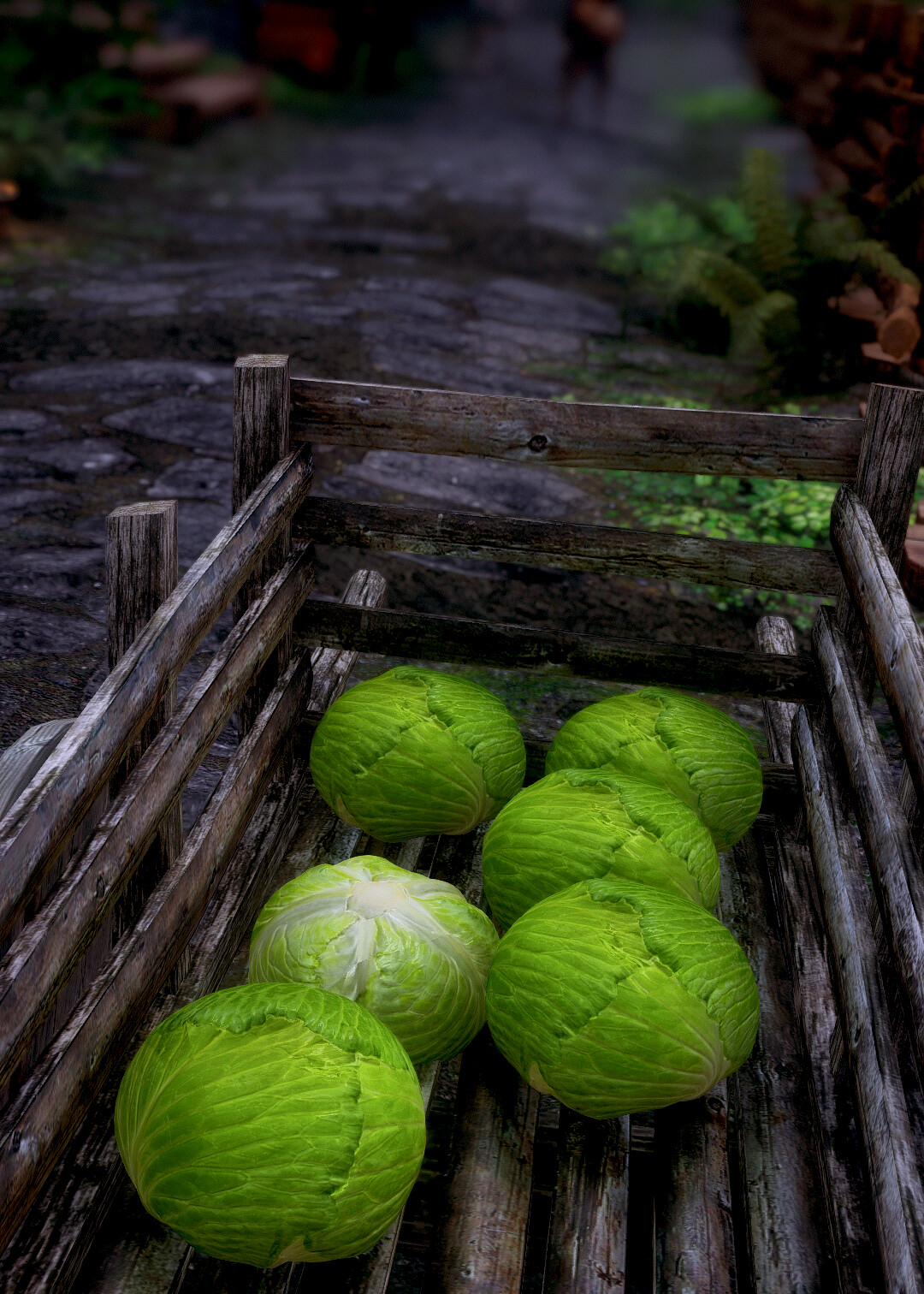The image depicts an old, rustic wooden container, reminiscent of something one might see in the past, possibly used for farming. Inside this well-worn wooden crate, there are six vibrant, green heads of lettuce. The wooden container features visible slats and appears to be placed outdoors on the ground. The heads of lettuce are neatly arranged, with one upside down, revealing its white veins and stem. The background of the photo is slightly blurry and seems to be dark and damp, suggesting it might have recently rained. Green vines and bushes can be seen in the backdrop, along with a stone or rock pathway, adding to the natural, garden-like setting.